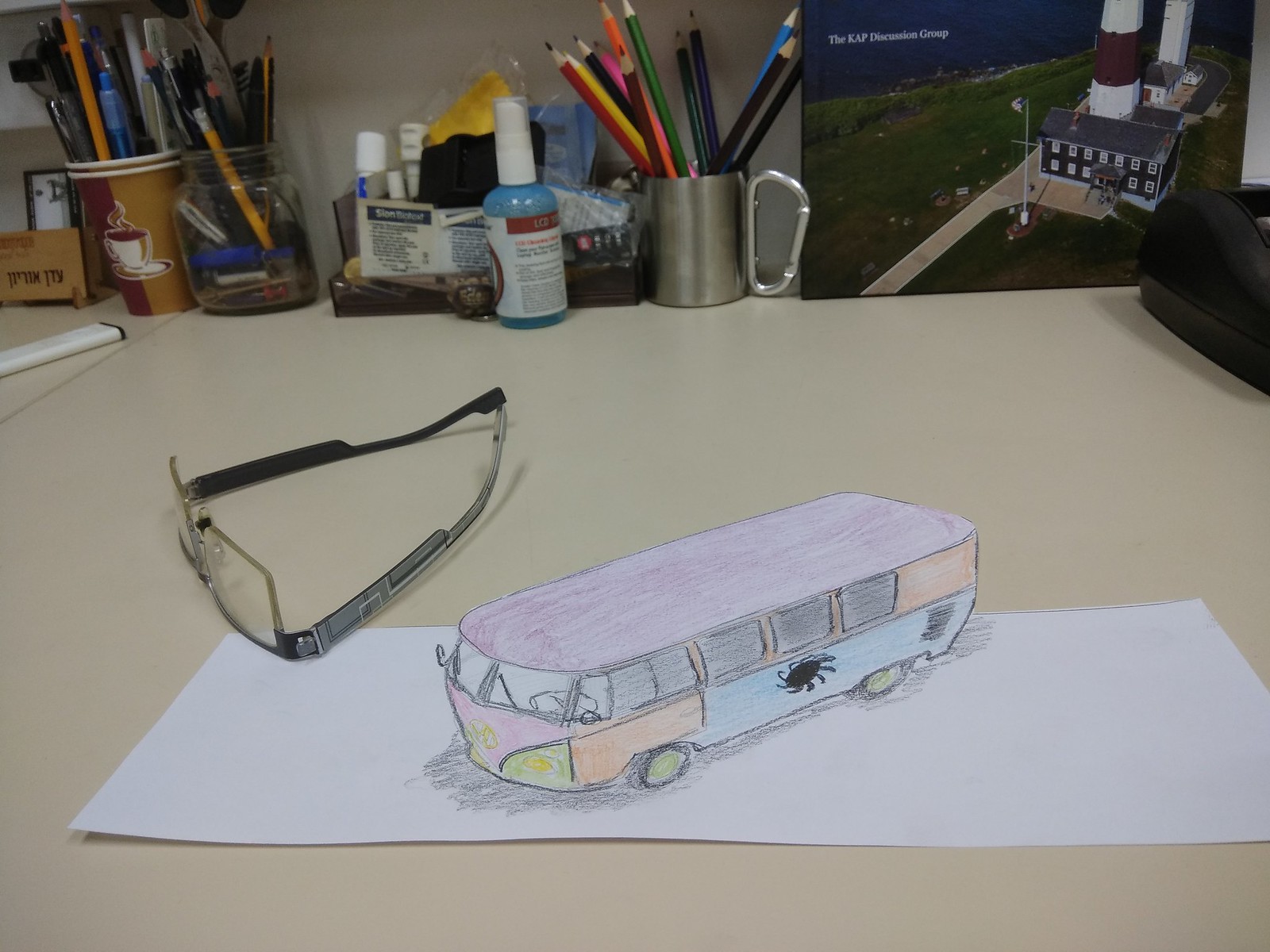A detailed, colorful drawing of the iconic Mystery Machine from Scooby-Doo is placed on a long flat piece of white paper, creating a three-dimensional illusion. The van is intricately colored with a light purple roof, light orange and blue sides, and neon green hubcaps. The front of the van has a light pink hue with light green and yellow accents where the headlights are. There are windows detailed along the side, and a black spider is drawn on the blue section, adding a whimsical touch. Near the paper, there are safety glasses laid out, and in the background, a cluttered desk is visible with various items. Among them, a white coffee cup filled with colored pencils, a small blue bottle with a white top, and a mason jar with more writing instruments can be seen. Also present are brown paper coffee cups with coffee cup illustrations, a ruler, and a book or object featuring a building and white writing on its cover.